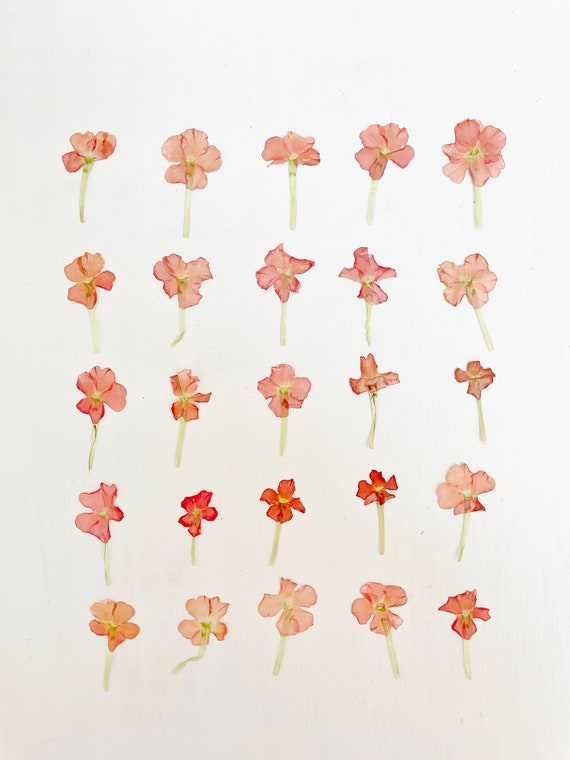The image depicts a watercolor painting of 25 flowers arranged in five horizontal rows, each containing five flowers. The background is a soft off-white or cream color, creating a gentle backdrop for the artwork. Each flower features about four to six petals with a color palette that ranges from a pinkish-red to a reddish-orange hue, accentuating their varied stages of bloom—some fully open, others more closed. The petals appear somewhat translucent, giving them a delicate, ethereal quality. In contrast, the flowers in the second to last row's center are more vividly colored, standing out with their solid appearance. The centers of the flowers are green, and the stems are a mix of brownish-green to watered-down green, with most being straight but a few slightly bent near the bottom. The simplicity of the arrangement and the lack of any additional elements like text or watermarks focus attention entirely on the floral display.